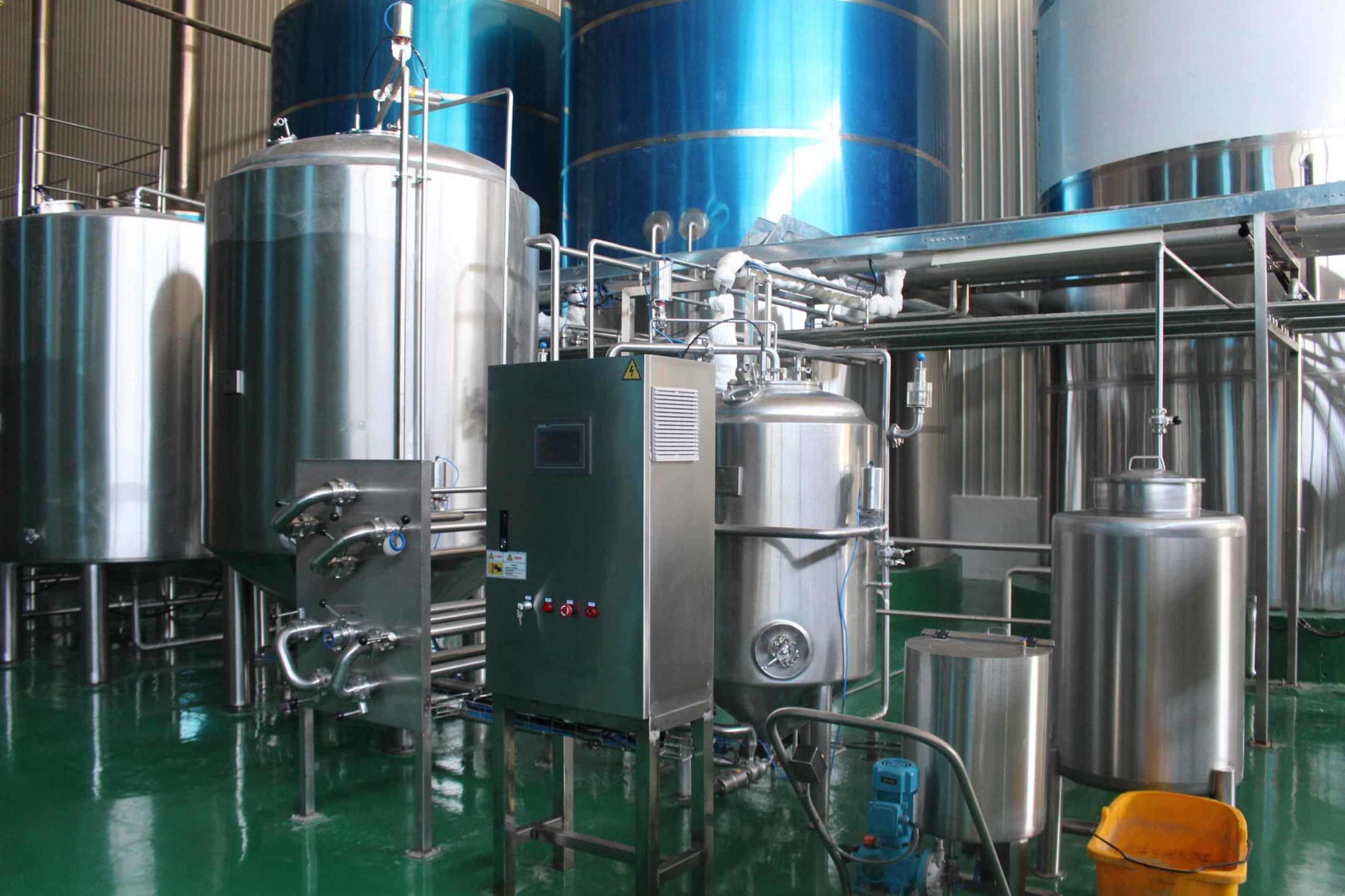This color photograph, reminiscent of a magazine feature, captures the intricate interior of an industrial plant, possibly a brewery. The image prominently displays an array of large, shiny silver canisters evenly spaced and accentuated by overhead lighting that highlights their metallic surfaces and various components. 

In the foreground, a yellow bucket sits in the bottom right-hand corner on a green ceramic-like floor, which reflects the light, adding to the metallic ambiance. Several of these silver canisters are mounted on steel beams, with knobs, valves, and handles visible on them, suggesting functionality in a processing setup. 

Behind these canisters stand two substantial blue cylindrical containers with silver trim, towering over the scene and adding a contrasting color to the predominantly grey setting. To the right, white rods emerge from a conductor box, and an electrical box with three red buttons and a security tag adds to the industrial complexity.

Piping runs between the canisters and the blue cylinders, indicating interconnectedness likely for fluid transfer. Each detail, from the silver legs of smaller canisters to the precise arrangement of metallic components, contributes to the sense of meticulous engineering. This highly detailed and reflective environment spotlights the technical and functional beauty of industrial design.